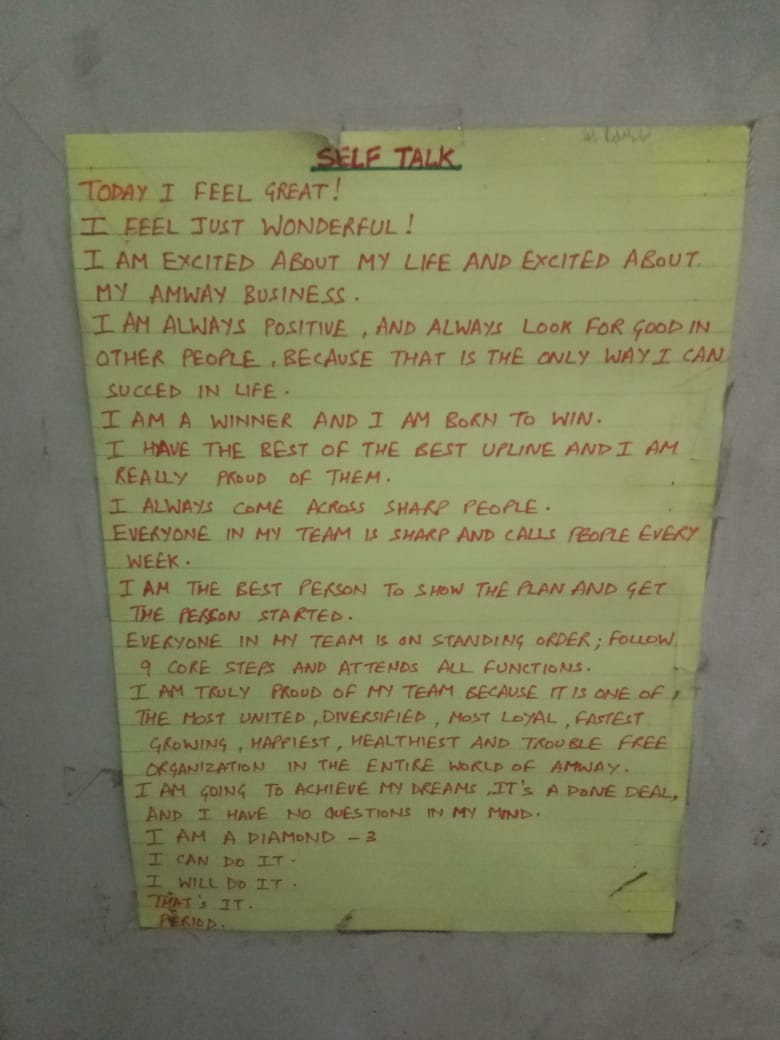The photograph captures a piece of yellow notebook paper taped to a dirty, smudgy white wall. The paper itself appears quite dirty as well. At the top, written in red ink and underlined, is the title "Self-Talk." Below this, the text continues in red ink, beginning with "Today I feel great. I feel just wonderful. I'm excited about my life and excited about my Amway business. I am always positive and always look for good in other people because that is the only way I can succeed in life. I am a winner and I am born to win. I have the best of the best upline and I am really proud of them. I always come across sharp people. Everyone in my team is sharp and calls people every week. I am the best person to show the plan and get the person started. Everyone in my team is on standing order, follows nine core steps, and attends all functions. I am truly proud of my team because it is one of the most united, diversified, the most loyal, fastest-growing, happiest, healthiest, and trouble-free organizations in the entire world of Amway. I am going to achieve my dreams. It's a done deal and I have no questions in my mind. I am a diamond. I can do it. I will do it. That's it, period." The note is covered in multiple lines of affirmations and motivational statements, culminating in a strong declaration of self-belief and commitment to success.